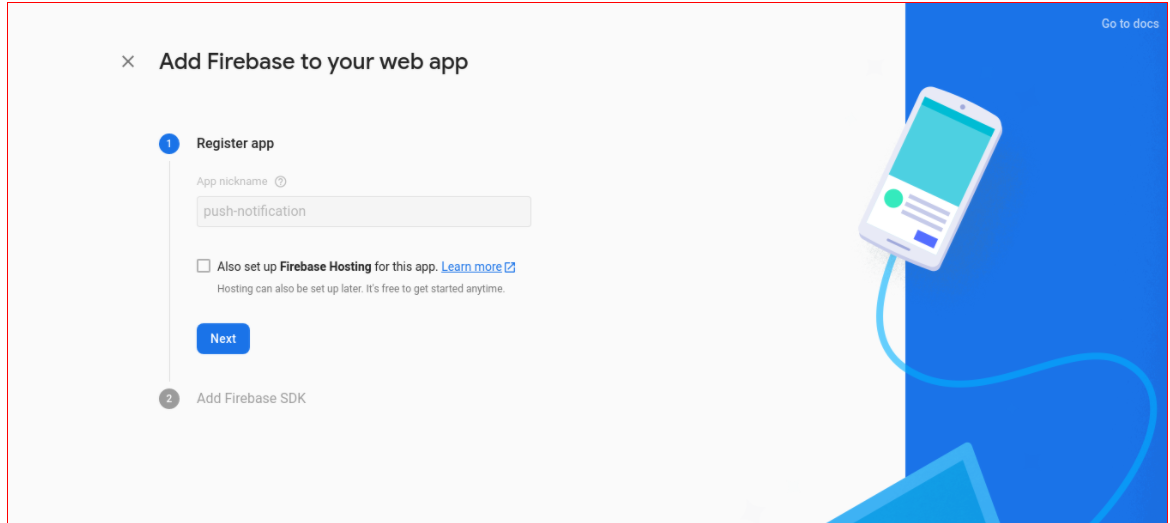The image displays a webpage dedicated to adding Firebase to a web application. In the top left corner, there's a header that reads, "Add Firebase to your web app." Underneath this header, the page is divided into various sections guiding the user through the registration process.

Just below the header, there is a section titled "Register App" which features an input field labeled "App nickname." This field allows users to enter a custom name for their application. An example nickname "Push Notification" is given, suggesting a potential function or feature of the app. 

Adjacent to the input field, there is a checkbox option that says, "Also set up Firebase Hosting for this app." Next to this option is a hyperlink labeled "Learn more," offering additional information on Firebase Hosting. Beneath this checkbox, a note states, "Hosting can also be set up later. It's free to get started at any time."

At the bottom of this section, a prominent blue button with white text labeled "Next" allows users to proceed to the next step.

The second step, "Add Firebase SDK," is mentioned below, indicating the progression of the setup process. On the right side of the page, there is an illustration of a smartphone connected by a blue cable. The screen of the smartphone is green and prominently features a bright green button, visually representing the interface of the application.

Overall, the webpage provides a structured and user-friendly interface to help users integrate Firebase services into their web applications.